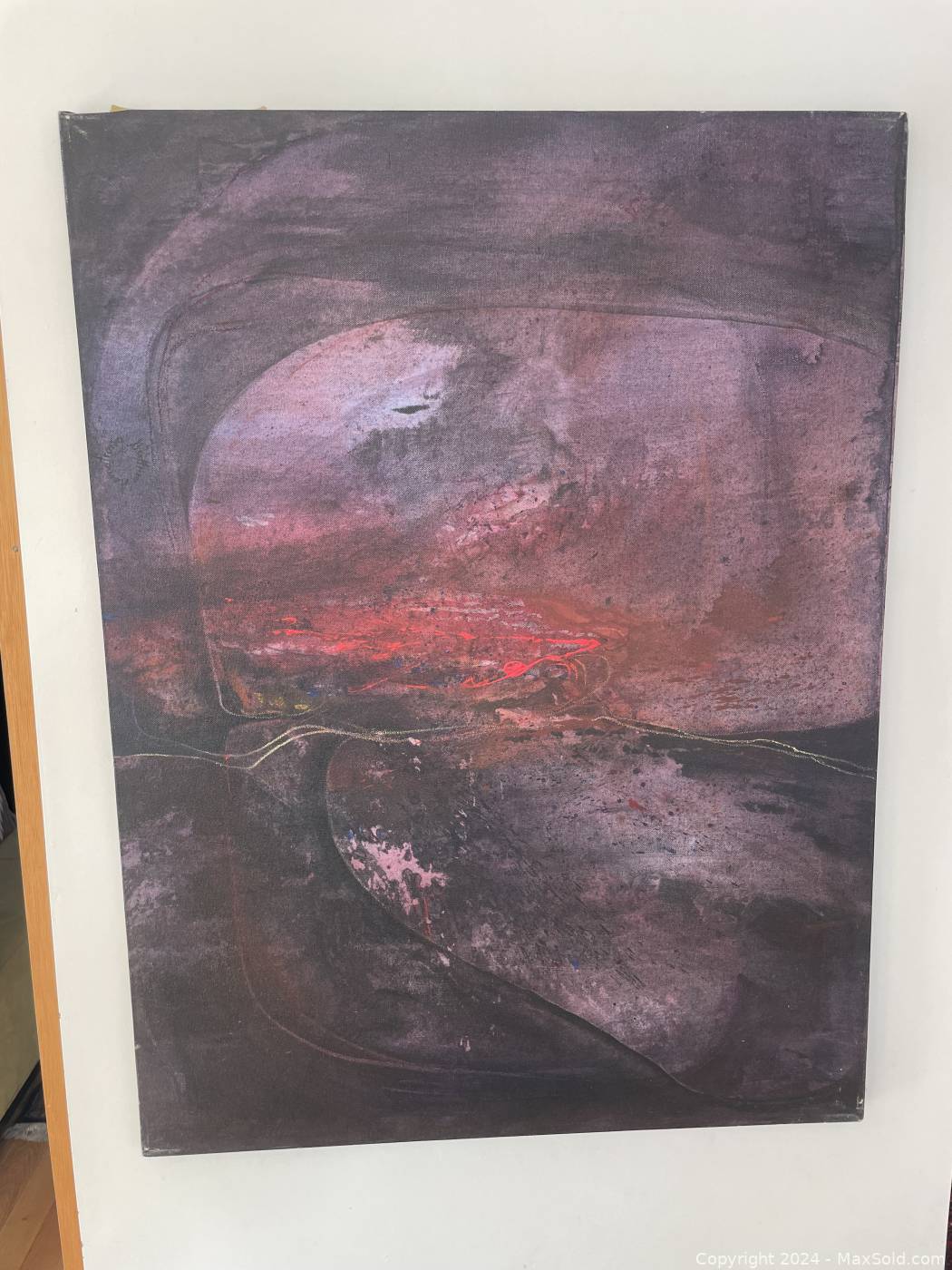This image is a painting encased in a thin, light-brown wooden frame with a white matte board border, standing on what appears to be a table or a wooden floor. The artwork itself is abstract, incorporating a variety of colors and encouraging personal interpretation. Dominant colors include black, gray, red, blue, and purple. The painting features a flowing composition from front to back. Some viewers might perceive elements resembling a natural landscape. There appears to be a red, lava-like flow suggestive of a volcanic eruption, with a potential mountain or volcano in the background. The upper portion has dark purple tones, hinting at a curved cave ceiling, while the bottom suggests a curved floor with what could be interpreted as a pink and black pool of water. The overall abstract nature leaves much to the viewer’s imagination, offering a visually intriguing experience.